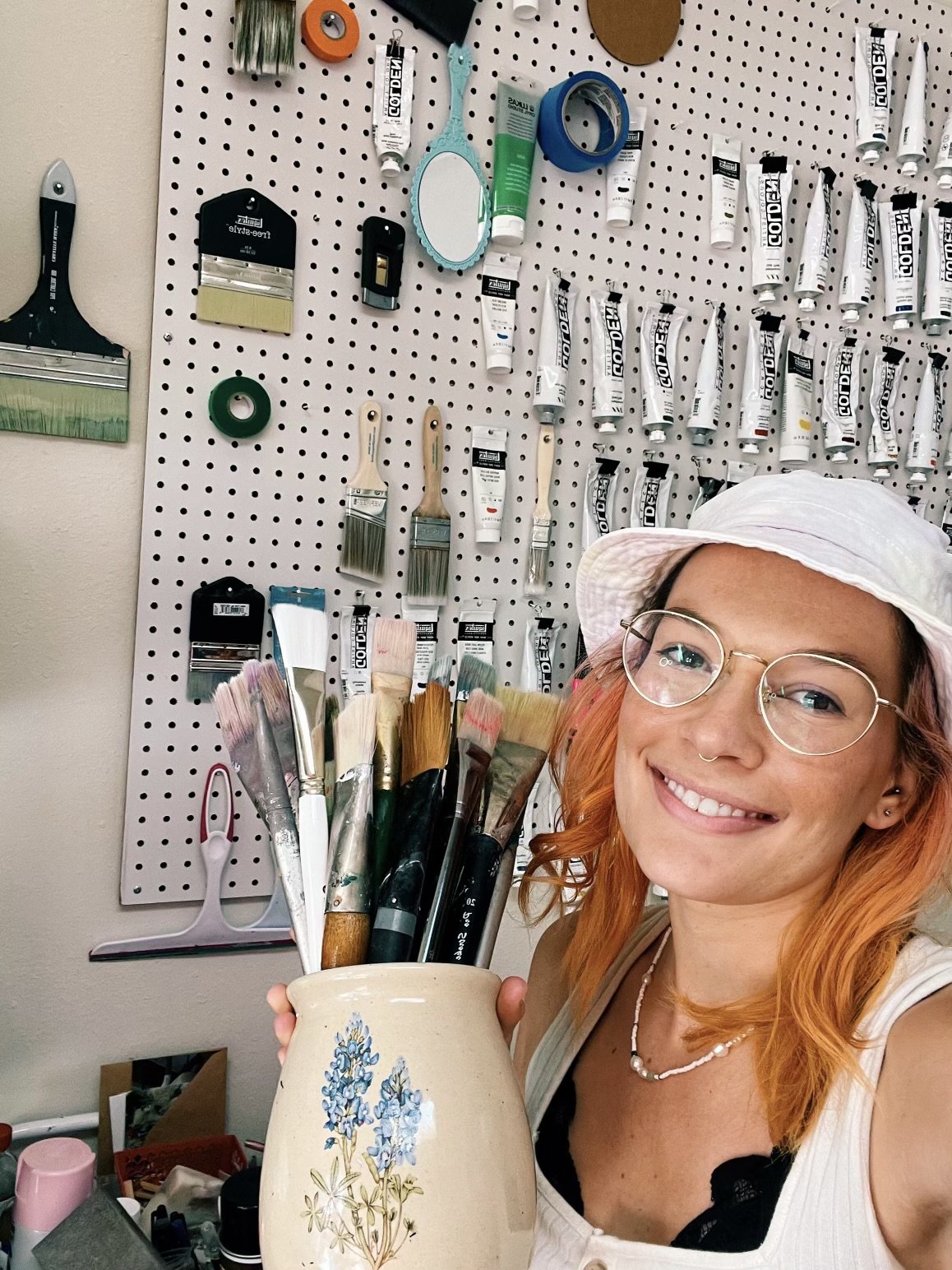In this indoor photograph, a smiling woman with orange-dyed hair is showcased from the waist up, wearing a white bucket hat, silver-framed glasses with clear lenses, and a white tank shirt with buttons down the front. She accessorizes with a necklace composed of white beads interspersed with white pearls and a small silver septum piercing. Cradling a cream-colored pot adorned with a flower design in her right hand, she proudly displays an assortment of paintbrushes of varying sizes and lengths inside the pot. Behind her, a white wall is adorned with numerous hanging paintbrushes, tubes of white paint, and a mirror. The woman's happiness radiates through her smile, making the scene both cheerful and artistically vibrant.